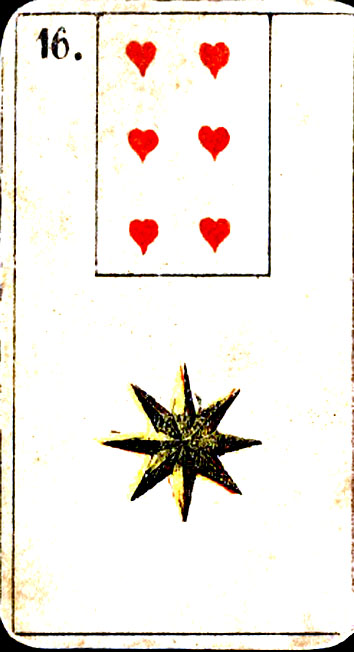The image depicts an intriguing card with characteristics reminiscent of both playing cards and tarot cards. This card has rounded edges and sits on a dark surface, making it stand out. The card features six red hearts arranged in two columns of three, creating a symmetrical pattern. In the upper left corner, there is the number "16" followed by a period, printed in black.

Surrounding the hearts is a rectangular border, similar to those found on traditional playing cards. Beneath this border, a large eight-pointed star, primarily black with yellow accents, dominates the lower portion of the card. The star’s design gives a subtle 3D illusion, enhancing its visual appeal.

The card’s background has an antiquated, weathered appearance, predominantly tan with patches that appear brownish, suggesting it is aged or has been handled frequently. This gives the entire image a vintage feel and adds to its mysterious allure. Despite its resemblance to a playing card, the unique elements and overall design suggest it might be something more enigmatic, perhaps a page from an old book or a tarot card.